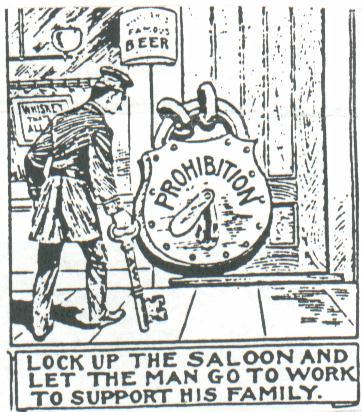The black-and-white cartoon drawing depicts a scene from the Prohibition era, likely from an old publication or advertisement of the time. In the center, a massive lock labeled "Prohibition" secures a wooden door, presumably of a bar or saloon. A person, probably a police officer, stands in front of it, holding a large key. Above the lock, the text "Famous Beer" is prominently displayed, and to the left, there is a window with a sign reading "Whiskey." The whole image exudes a simplistic, comic book style, with a slight crookedness that suggests it may have been scanned from an older source. Below the drawing, a caption in capital letters reads, "LOCK UP THE SALOON AND LET THE MEN GO TO WORK TO SUPPORT HIS FAMILY," underscoring the Prohibition message encouraging men to leave bars and focus on supporting their families through work.